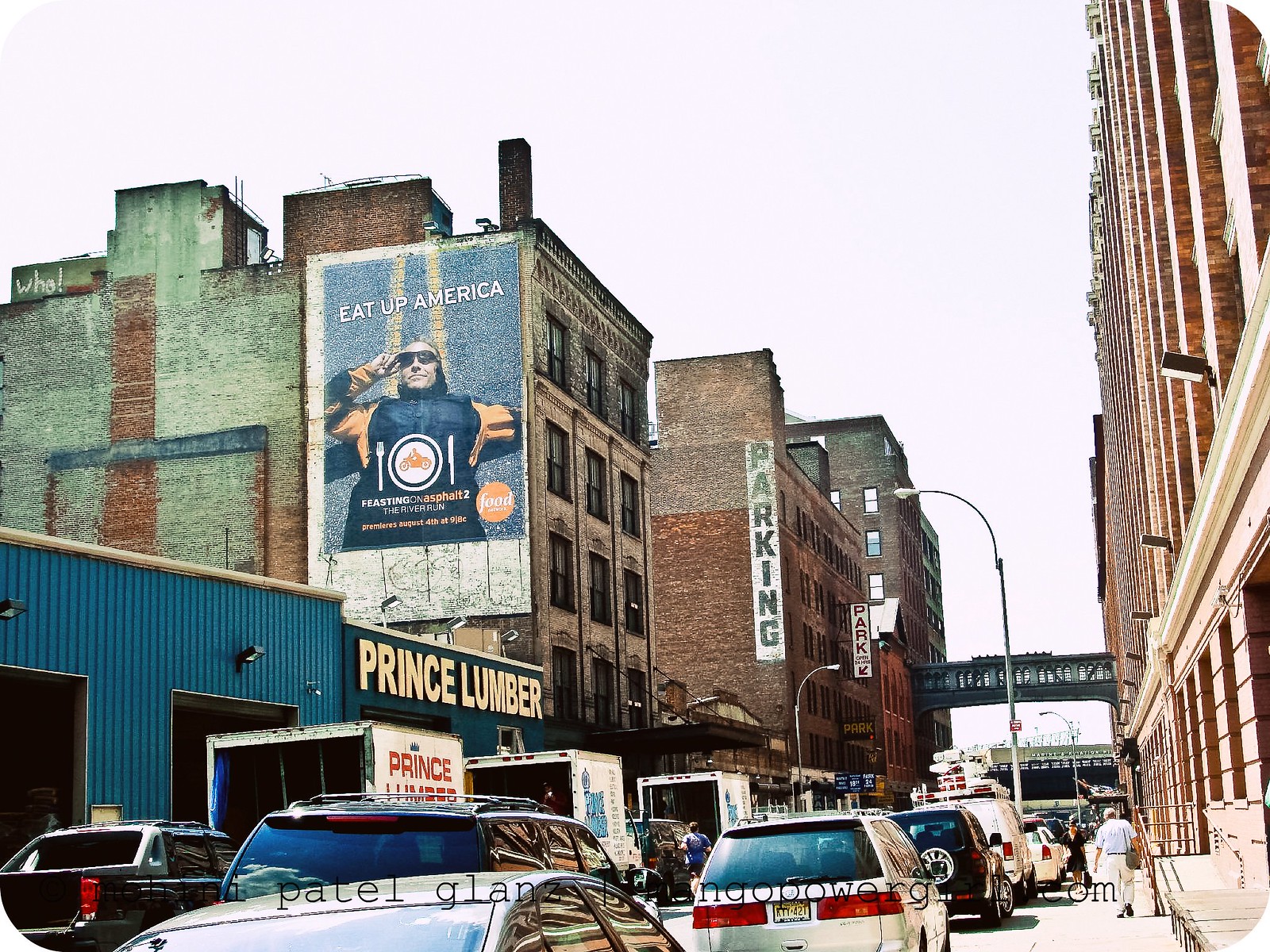This image captures a bustling city street in an old, brick-laden downtown area under a light white-blue sky. Prominently on the right, there is a blue aluminum-sided building labeled "Prince Lumber" with open garage doors and several white moving trucks displaying the same name parked in front. Adjacent to it is a large, brown-brick building adorned with a billboard that reads "Eat Up America" along with "Feasting on Asphalt 2, the River Run" and the Food Network logo. The billboard features a man in sunglasses lying on road stripes with a plate bearing an orange motorcycle and utensils. This building has a brown facade, extends four stories high, and follows a pattern of three windows per story. Further down, a series of other old, red and dark brown brick buildings, including a parking garage with a bridge connecting two structures, line the street. On the left side of the road, there is a sharp view of the buildings due to the camera angle, with details such as a gentleman in a blue shirt and white pants walking, carrying a shoulder bag, and a woman in a dress up the street. Numerous cars, including a gray one, a black one, a white van, and another white car, are parked along the side of the road. At the bottom of the photo, there is a watermark that somewhat reads "Patel Glanz" and another indistinct word, suggesting a possible credit or ownership mark.